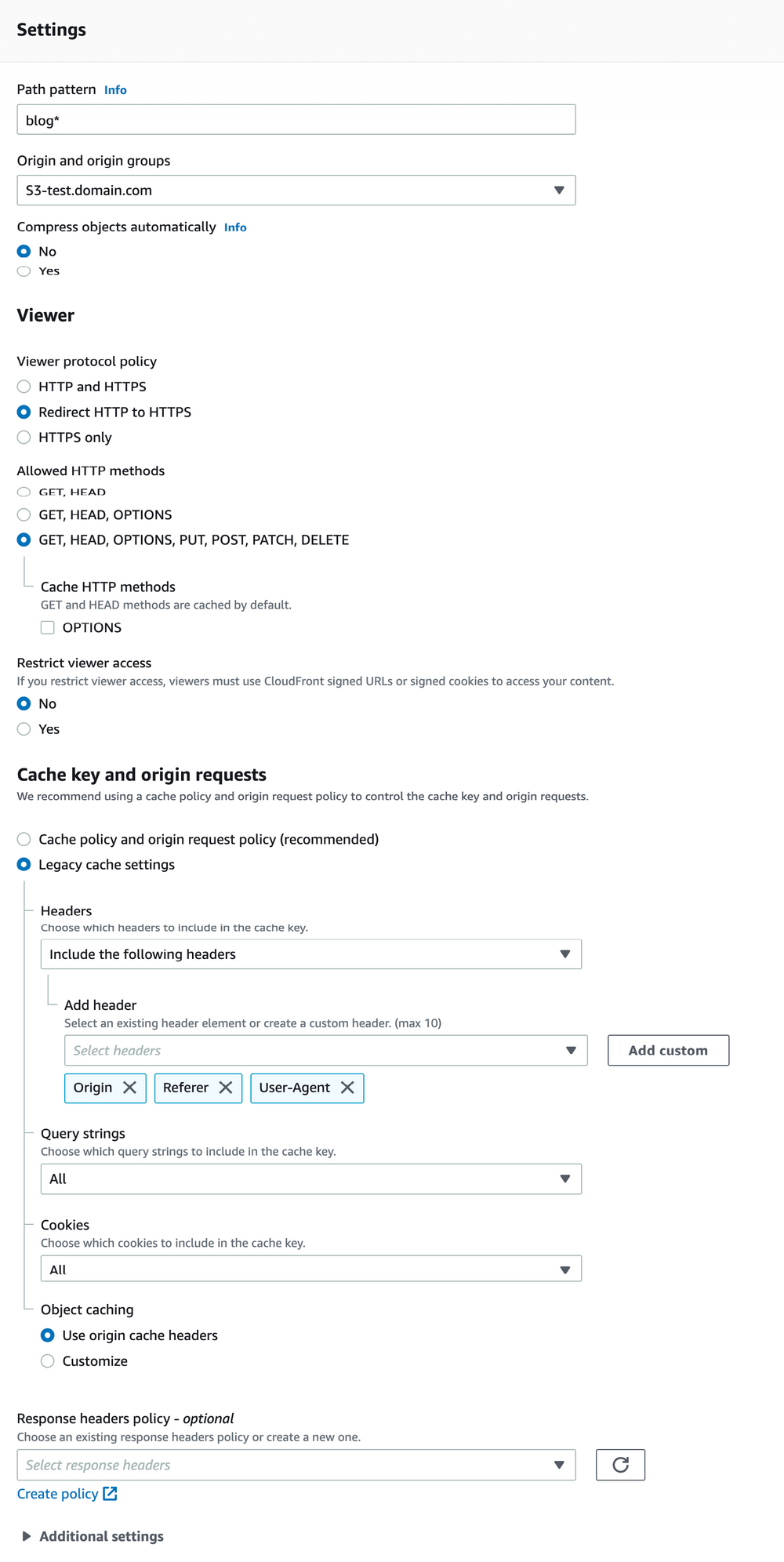This is a screenshot of a detailed settings page. At the very top, there is a grey bar with the word "Settings" displayed prominently on the top left. Immediately below, the first section labeled "Path Pattern" displays a text box containing the entry "blog*". Adjacent to this, there is an option labeled "Hide."

Following this, the next section is titled "Origins and Origin Groups." Here, there is a drop-down menu that has the selection "sitestdomain.com." 

Moving down, we encounter the "Compress Objects Automatically" setting, which has an information icon in small blue letters to its right. The current selection for this option is set to "No."

The next prominent heading is "Viewer." Under this section, the "Viewer Protocol Policy" is detailed. Among the three available options, "Redirect HTTP to HTTPS" is selected. Below this, the "Allowed HTTP Methods" section details the selected options, which include "GET, HEAD, OPTIONS, PUT, POST, PATCH, and DELETE." This is followed by "Restrict Viewer Access," which is currently set to "No."

The final category towards the bottom of the page is "Cache Key and Origin Requests." Here, "Legacy Cache Settings" are selected. Within this section, there is a subsection titled "Headers." This contains a drop-down menu where "Include the following headers" is selected. An "Add Header" drop-down menu is available, with a custom button labeled "Add Custom" to the right. Underneath, three specific tags are selected.

Further down, the "Query Strings" option is detailed, with the drop-down until set to "All." Similarly, the "Cookies" drop-down is set to "All." Lastly, the "Object Caching" setting states "Use Origin Cache Headers," which is selected by default.